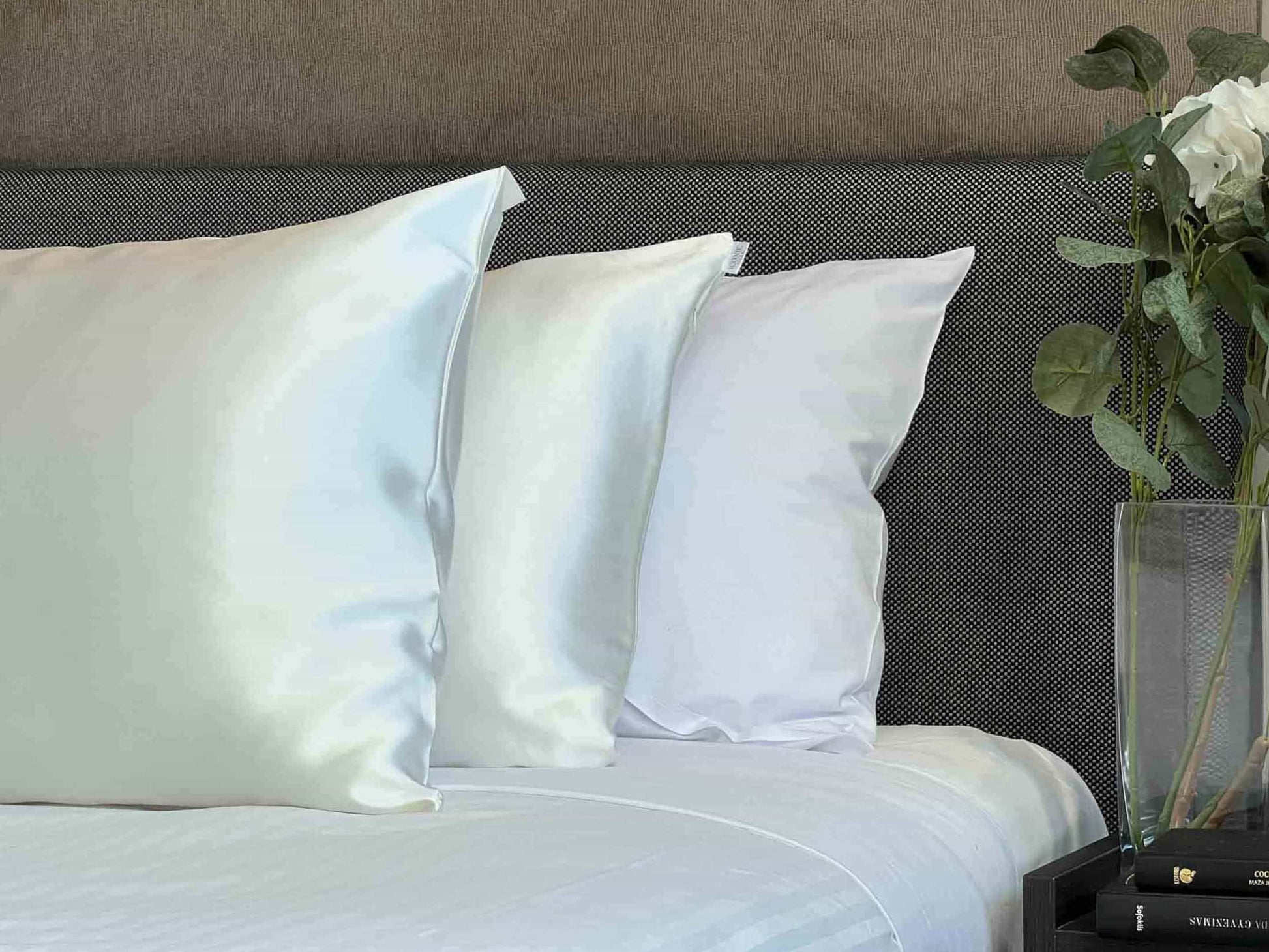The image depicts a serene bedroom setting, possibly in a hotel. Centered, there is a bed with neatly arranged white sheets featuring subtly shiny white stripes. The sheets appear to be satin and are elegantly folded down. Three pillows are neatly stacked on the bed; the two front pillows are covered in satin or silk pillowcases and are beneficial for hair, while the back pillow, which is resting against the headboard, has a cotton pillowcase.

The headboard is prominently black with a pattern of white dots and spans from the left to the center of the bed. Above the headboard is a wall that appears to be coated with a touchable, fabric-like, gray wallpaper, described by some as a light brown or taupe color. 

To the left of the bed stands a sleek black nightstand. Atop the nightstand are two black books and a tall, clear vase containing fake white flowers and green leaves, hinting at an artificial rose. The overall ambiance suggests a clean, orderly, and inviting space, typical of a refined hotel room.